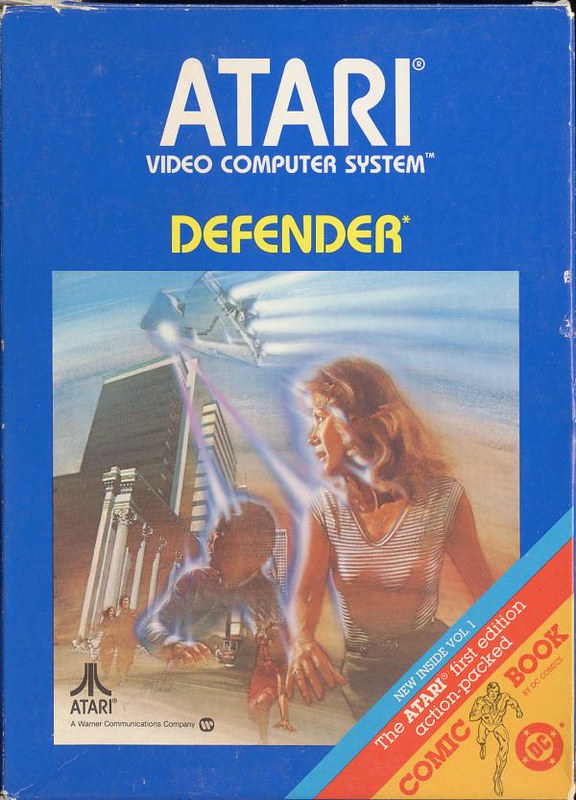The image features an Atari game box for the game "Defender." The top section of the box showcases a blue background with "ATARI" prominently displayed in large, white capital letters. Just below, “Video Computer System” TM is written, also in white letters. Beneath a space, the game's title "Defender" appears in bold yellow letters.

In the bottom right corner, a diagonal label stands out with multicolored sections: a blue stripe stating "NEW INSIDE VOLUME 1," an orange stripe declaring "THE ATARI FIRST EDITION ACTION-PACKED," and a yellow triangle marked with “COMIC BOOK” in bold. Adjacent to this is the text “BY DC COMICS” along with a depiction of a Superman-like character running towards the viewer, encapsulated in a red circular logo with a yellow inner circle and "DC" written in red inside it.

The bottom two-thirds of the box feature a dynamic illustration related to the "Defender" game gameplay. At the lower left corner of this section, "ATARI A WARNER COMMUNICATIONS COMPANY" is inscribed in black. The artwork prominently displays a woman in a sleeveless, v-neck striped shirt facing forward, though her gaze is directed to the left. Behind her, the torso of a man is visible, also looking in the same direction. In the sky, a spaceship firing lasers and a towering building they seem to be focused on are illustrated, adding an action-packed atmosphere to the scene.